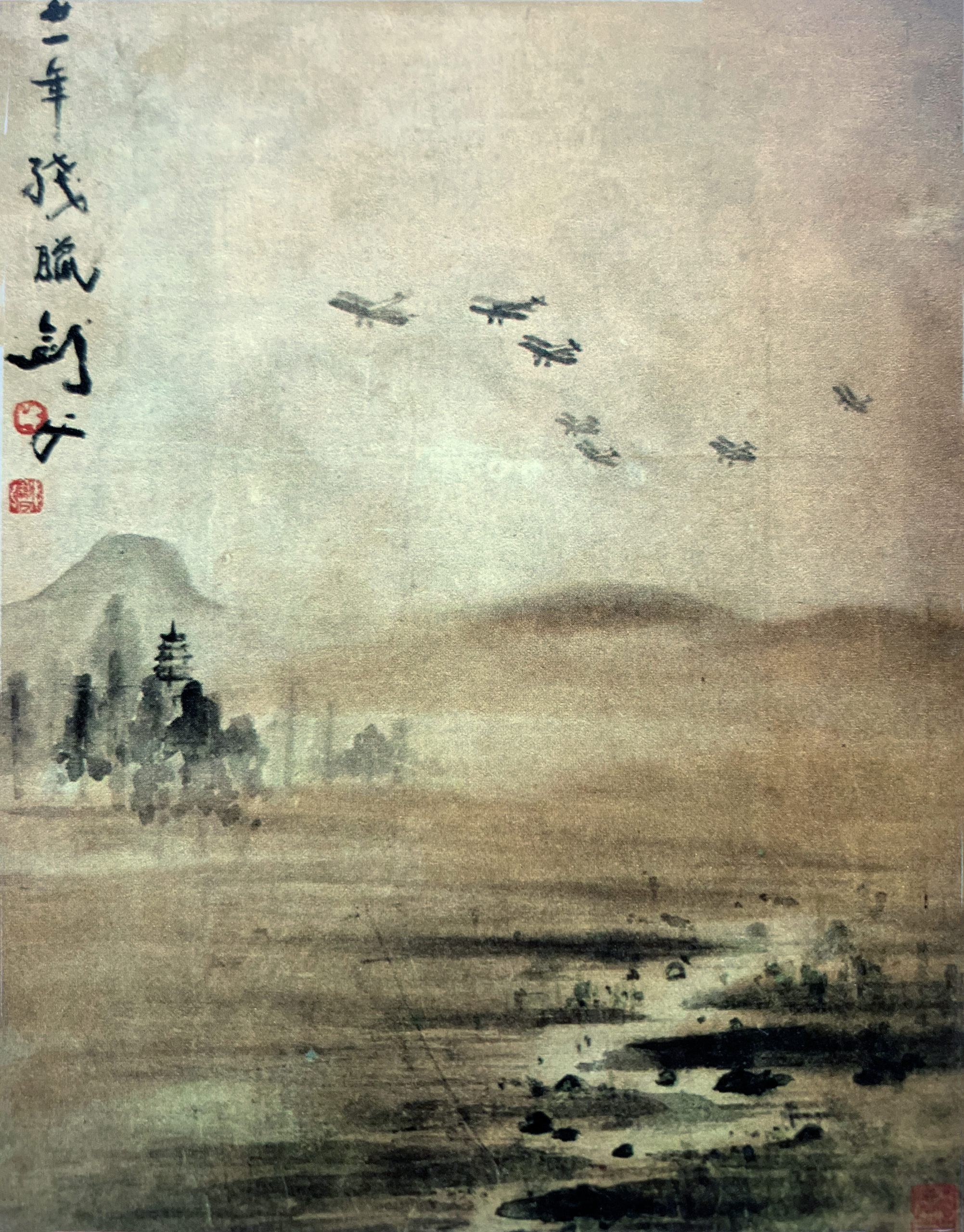This vintage Asian artwork, likely produced by a Chinese or Japanese artist, is a rich and detailed silk painting or lithograph. The sky features seven warplanes flying amidst a watercolor wash of bluish, taupe, and gray hues. The top-left corner of the artwork displays six large Asian characters, possibly Chinese, descending downward, accompanied by two red stamp seals, with another stamp seal in the lower right believed to mark the artist's identity. Below the planes, the distant hills and mountains are depicted in light brown and taupe colors, suggesting a desert landscape. In the background, there is a notable mountain with a plateau alongside softer, rolling hills. To the left, subtle, sweeping pine trees and other foliage, painted in black watercolor, add texture and depth. The foreground of the piece features a mix of brown, taupe, ivory, and black horizontal lines, accented with dots that suggest stones and a pond or creek, giving the scene an added layer of richness and subtle movement.